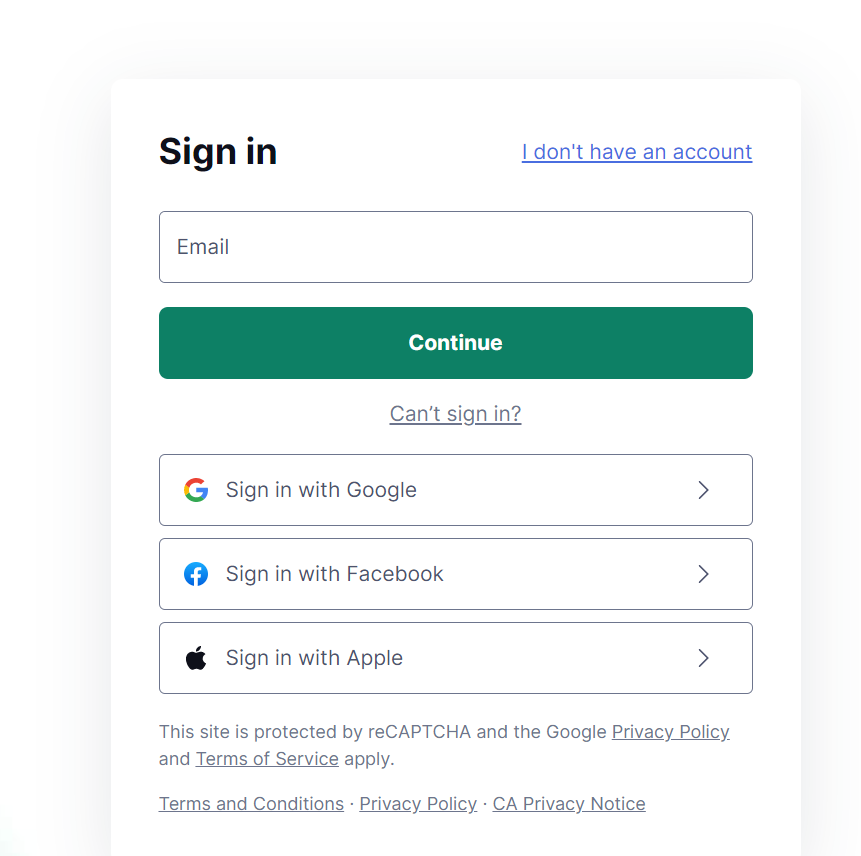The image depicts a website's sign-in page. Dominating the center is the "Sign In" option. To the right, there's a blue, underlined link labeled "I don't have an account" for new users. Below, there's a field for email input. If users can't sign in with their email, they are presented with alternative options to sign in using Google, Facebook, or Apple, each accompanied by their respective symbols and dropdown menus, though none of these menus are currently expanded in the image. 

At the bottom, a note indicates that the site is protected by reCAPTCHA, and links to the Google Privacy Policy and Terms of Service are provided. Additional clickable links for "Terms and Conditions," "Privacy Policy," and "California Privacy Notice" are also available. The text on the page is predominantly in black font with varying sizes on a white background. Ellipses are present, highlighting areas related to the alternate sign-in methods. Finally, a prominent green button labeled "Continue" invites users to proceed if they agree with the site's terms.